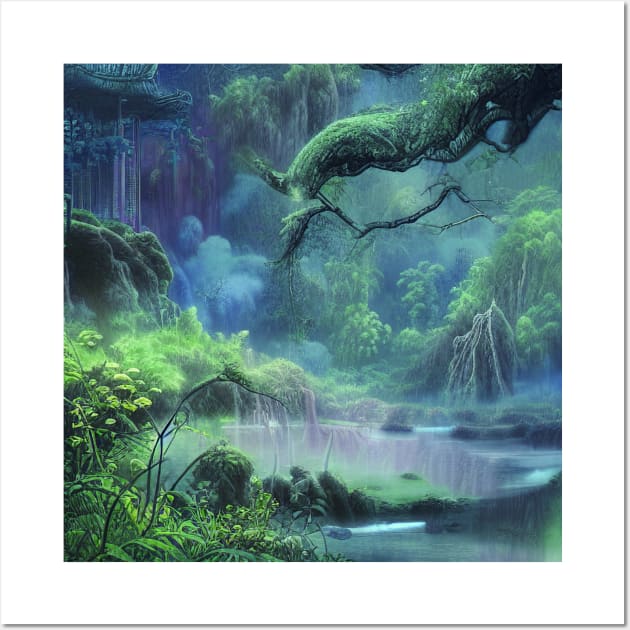This detailed, fantasy-like painting, rendered in soft acrylic tones, captures an enchanted forest scene at what appears to be nighttime or under dense tree cover. The focus is a misty, swamp-like pond at the center, surrounded by lush, vibrant green vegetation and moss-covered rocks. The forest is depicted with a variety of large trees, overhanging branches, cliffs, and hills, all adorned with moss. In the distance to the left, there seems to be a structure resembling a temple with a thatched roof, although it's partially obscured and could blend with the dense foliage. Puffy clouds can be faintly seen in the background, adding to the mystical ambiance. The entire scene is enveloped in a foggy haze, enhancing its otherworldly and serene atmosphere. No text or signature is present on this captivating piece, which beautifully encapsulates the essence of a mystical, tropical forest.